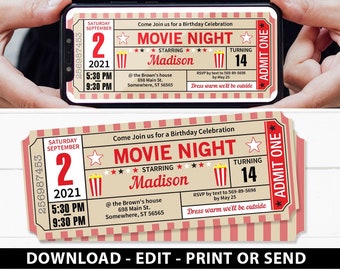The image is a detailed montage showcasing custom movie ticket-style invitations for a birthday celebration. At the top, a photograph captures a man's hands presenting a personalized movie ticket amid a partially cropped, undefined background. This ticket highlights a 2021 birthday event for Madison, who is turning 14, with the party scheduled from 5:30 to 8:30 pm in February. Below, a close-up shows the same ticket design laid flat against a white surface, surrounded by additional tickets. The vibrant color scheme consists of pink, flesh tones, dirty yellow, white, and black. A banner at the bottom instructs viewers to download, edit, print, or send these creative invitations, emphasizing their versatility and the unique approach to inviting guests.